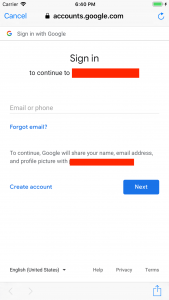The image depicts a smartphone screen displaying a slightly blurred Google account sign-in page under the category Websites. At the top of the screen, the status bar shows "Carrier" with Wi-Fi connectivity indicated. The time on the screen is too blurry to discern, but the battery icon is green and full. The header of the page features a blue "Cancel" option, a lock icon, and the URL "accounts.google.com", along with a refresh button. Below that, there is the familiar Google "G" logo followed by the text "Sign in with Google."

The phrase continues with "Sign in to continue to", but the word "to" is obscured by an orange line rather than black. Beneath this, users are prompted to enter their "Email or phone." In blue text just below, there is an option to "Forget email." A notification then indicates, "To continue, Google will share your name, email address, and profile pictures with", followed by more text obscured by a black line. Further down, the screen features "Create account" and a blue "Next" button. The footer of the page displays links to "English," "Help," "Privacy," and "Terms."